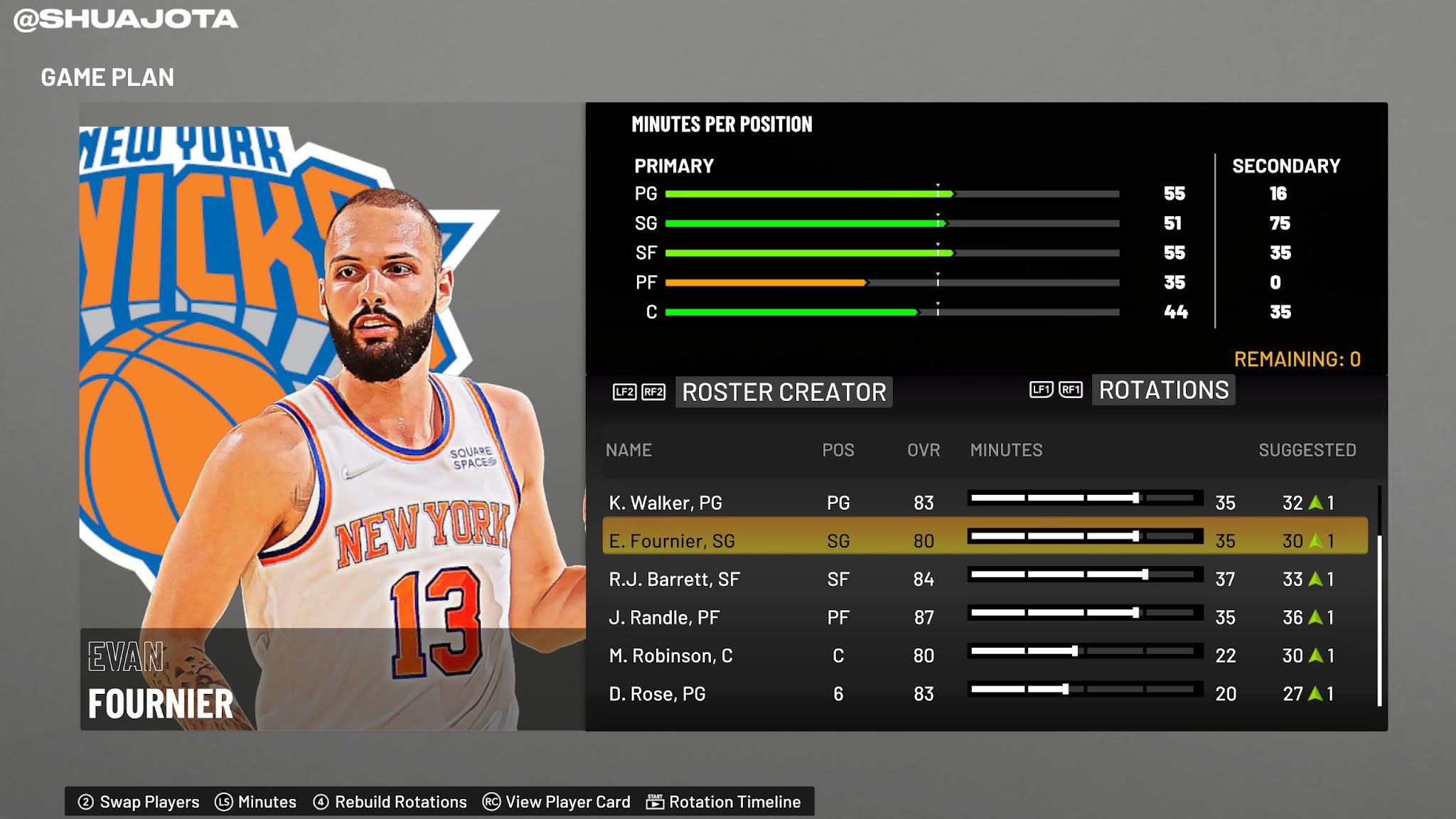The image displays a detailed web page showcasing player statistics for an American NBA basketball player. The background is grey with white text, and there is an inset square about 5% in from each side. This square is divided into two sections. On the left side, which occupies approximately 25% of the square’s width, there is a large hero image of the basketball player. The background features the New York Knicks logo, with the player standing in front of it, wearing a New York Knicks jersey bearing the number 13. At the bottom of this section, the player's name, Evan Fournier, is prominently displayed.

On the right side of the square, occupying about 75% of the space, various player statistics are displayed. These stats include minutes played per position, listed as PG (Point Guard), SG (Shooting Guard), SF (Small Forward), PF (Power Forward), and C (Center). The respective minutes for each position are 55, 51, 35, 35, and 44.

Below the statistics is a section labeled "Roster Creator." Evan Fournier is selected as part of the roster, and there are additional players listed, indicating that this feature may be used for a game where players can select different team members to assemble their ideal team.